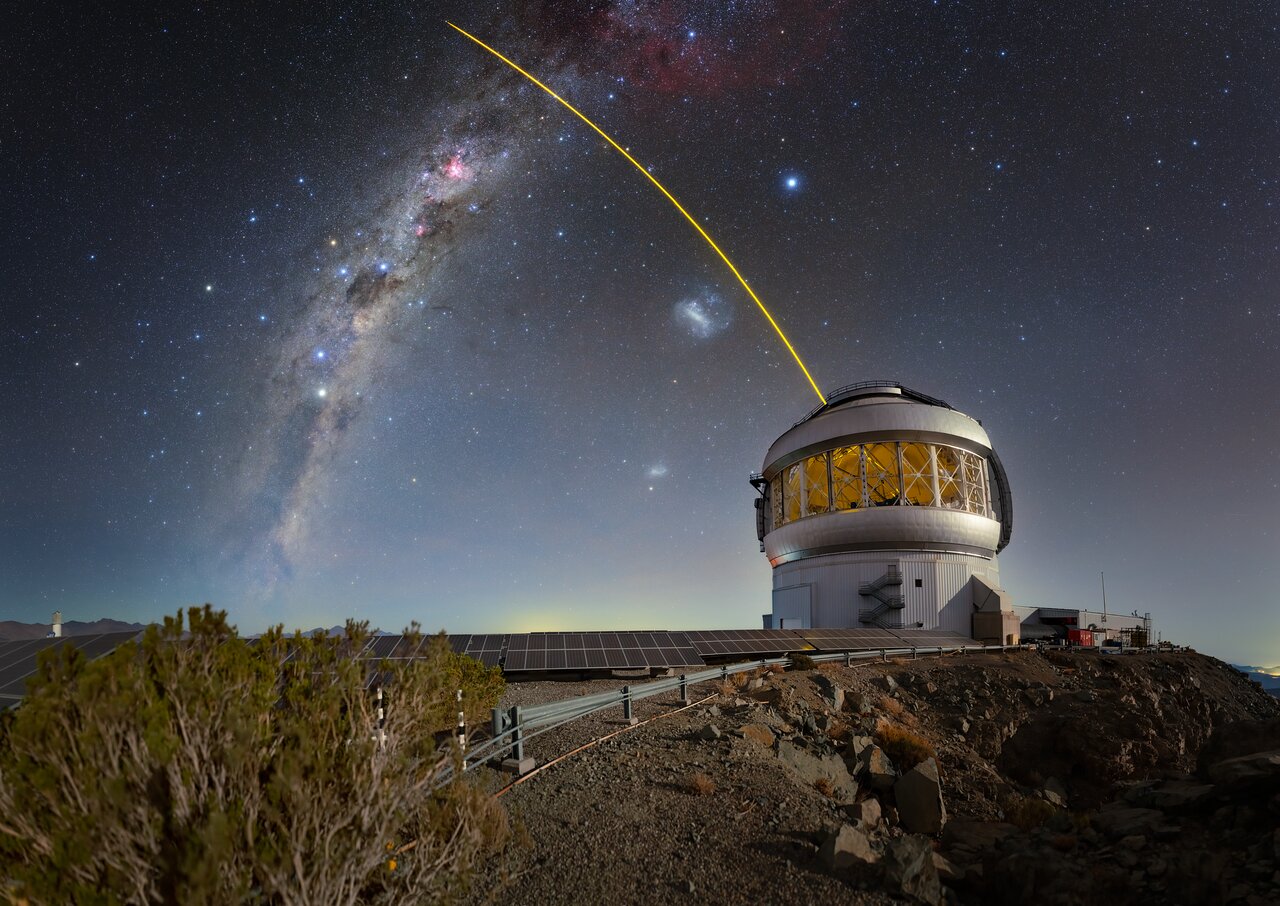This color photograph captures a serene nighttime scene featuring a dome-shaped observatory perched atop a hilly mountain. The dark blue sky, tinged with light hues of blue and pink, is adorned with numerous bright stars and a prominent, galaxy-like structure that stretches from the top to the bottom of the image. The observatory itself is a metallic gold or silver color with glass windows encircling its middle, and a metal staircase leading to a second-floor door. A striking yellow laser-like beam arcs out of the observatory's dome, curving towards the center top of the image. The foreground of the image is populated with solar panels stretching across the terrain, leading up to the observatory, accompanied by rocky outcrops and patchy green vegetation. The scene is further enhanced by a small building to the right of the observatory and a guardrail surrounding a rocky area on the far right.